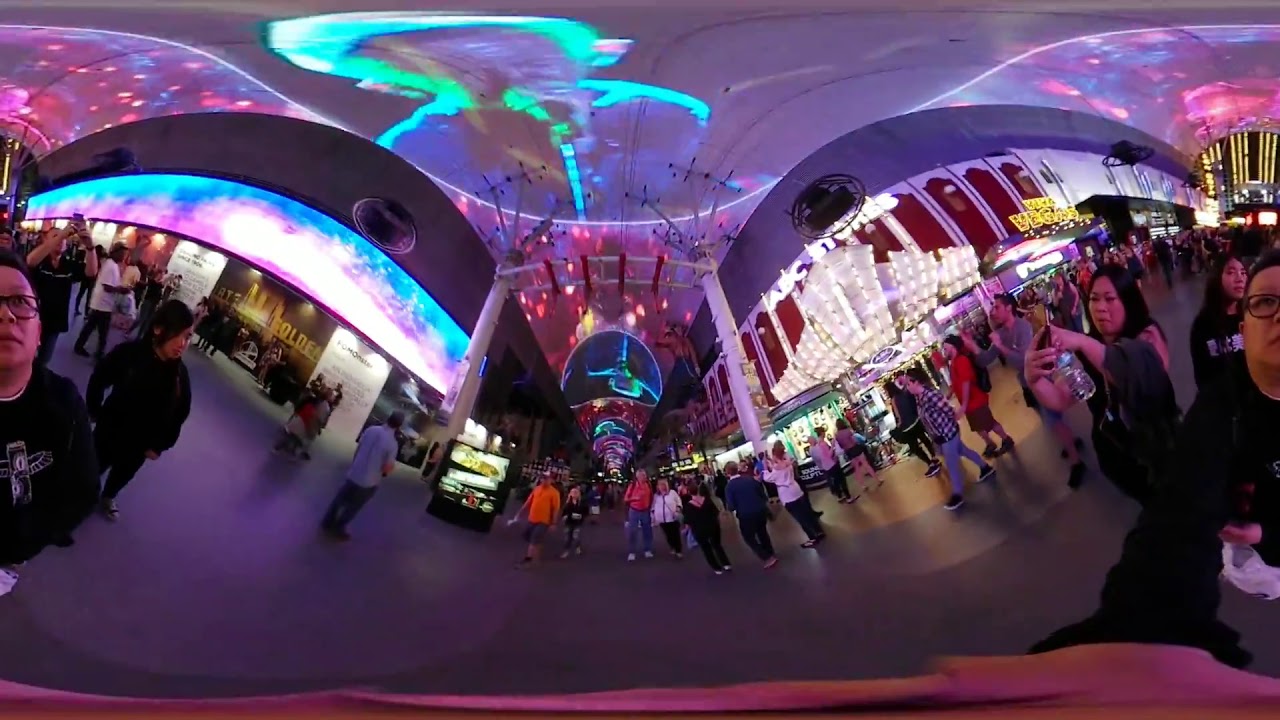The image portrays a vibrant and bustling scene at an indoor shopping mall, likely located in an Asian country. The photo, which appears to be a 360-degree panorama, captures a large crowd of people walking around and taking pictures with their camera phones. The ground is smooth, resembling polished concrete. The scene is filled with commercial facilities, including shops and possibly restaurants, with numerous lights adorning the ceiling. Blue waves and pink and red fireworks are colorfully projected overhead. 

In the foreground, the image’s panorama effect causes a distortion, making objects on either side appear bent. For instance, on the right side, there's a brightly lit sign that reads "ABC Stores," while the left side showcases a storefront with blue, pink, and white rainbow hues. Amid the crowd, a notable figure—a female wearing glasses looking up—is visible on the very edge of the photograph. There is a rich palette of colors throughout the image, including red, purple, black, white, tan, blue, light blue, green, and yellow, enhancing the dynamic and lively atmosphere.